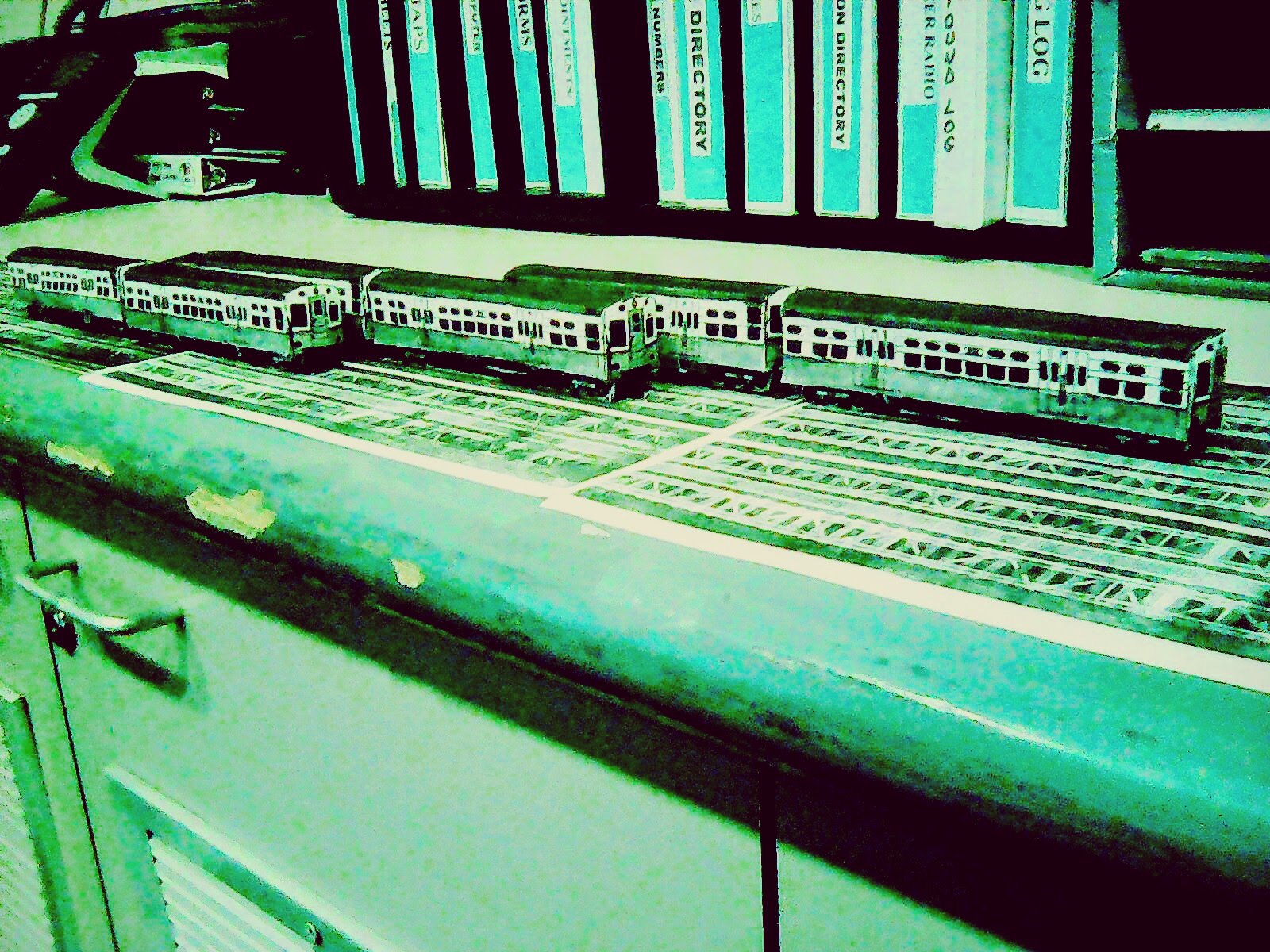The photograph depicts a room with an industrial or factory aesthetic, heavily filtered in shades of green, giving it a distorted, monochromatic effect. The primary subject is a countertop that appears well-worn and scuffed, positioned above cabinet doors with metallic D-shaped handles and what looks like a locking mechanism. Sitting on the countertop are six model passenger train cars arranged in three rows of two. These trains rest on sheets of paper designed to resemble train tracks. Scattered beneath the model trains are photographs, seemingly serving as references for detailing the model trains, which prominently feature green and white colors with detailing like windows. Behind this scene, there is a shelf filled with books or possibly directories and logs, including one clearly marked "LOG" and others labeled "DIRECTORY". The lower half of the books is visible, displaying black capital letters on a teal or turquoise background. The image has a grainy texture coupled with the green hue, contributing to its vintage or industrial ambiance.